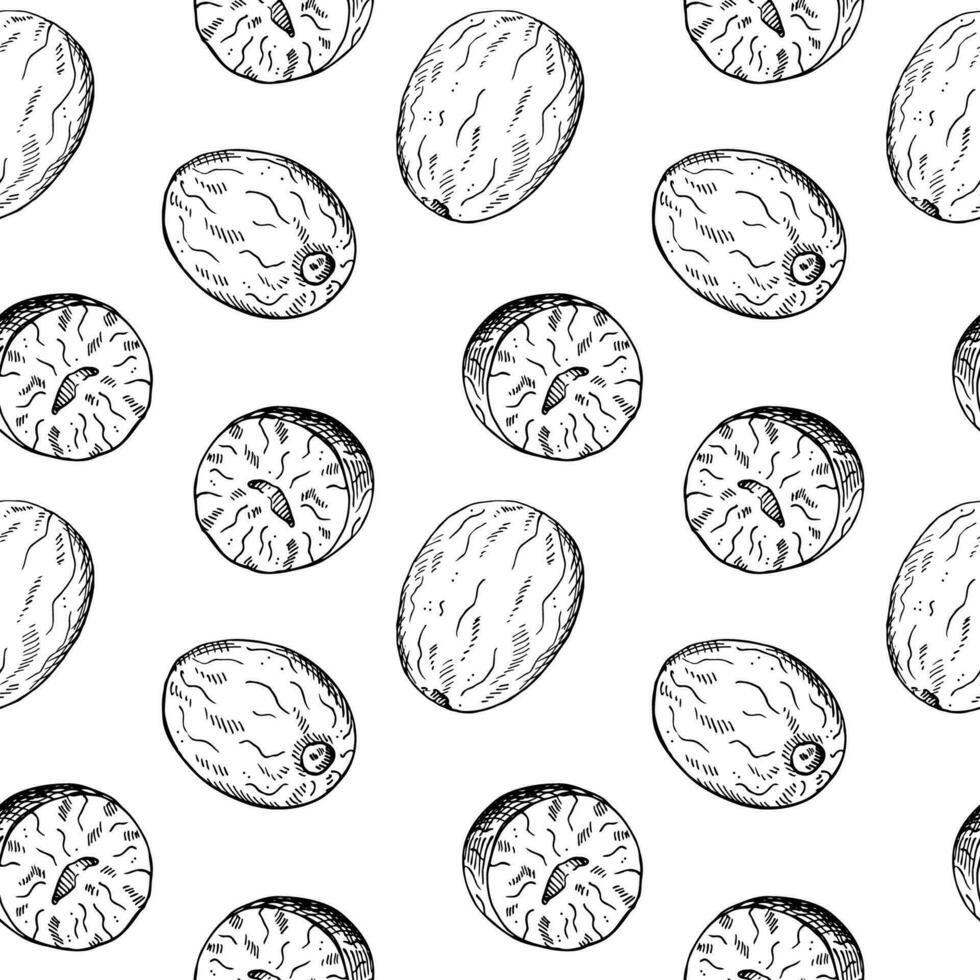This is a detailed black-and-white pencil sketch depicting numerous nutmegs against a white background, resembling an artistic wallpaper. The nutmegs are illustrated in various states: some are whole, while others are cut in cross-section showcasing their intricate inner structure. Each whole nutmeg features a small hole at one end, while the cut ones reveal a crescent-shaped worm-like pattern at their cores. The sketches use fine lines and short shaded strokes to add texture and depth, creating a simple yet expressive representation of the spice.